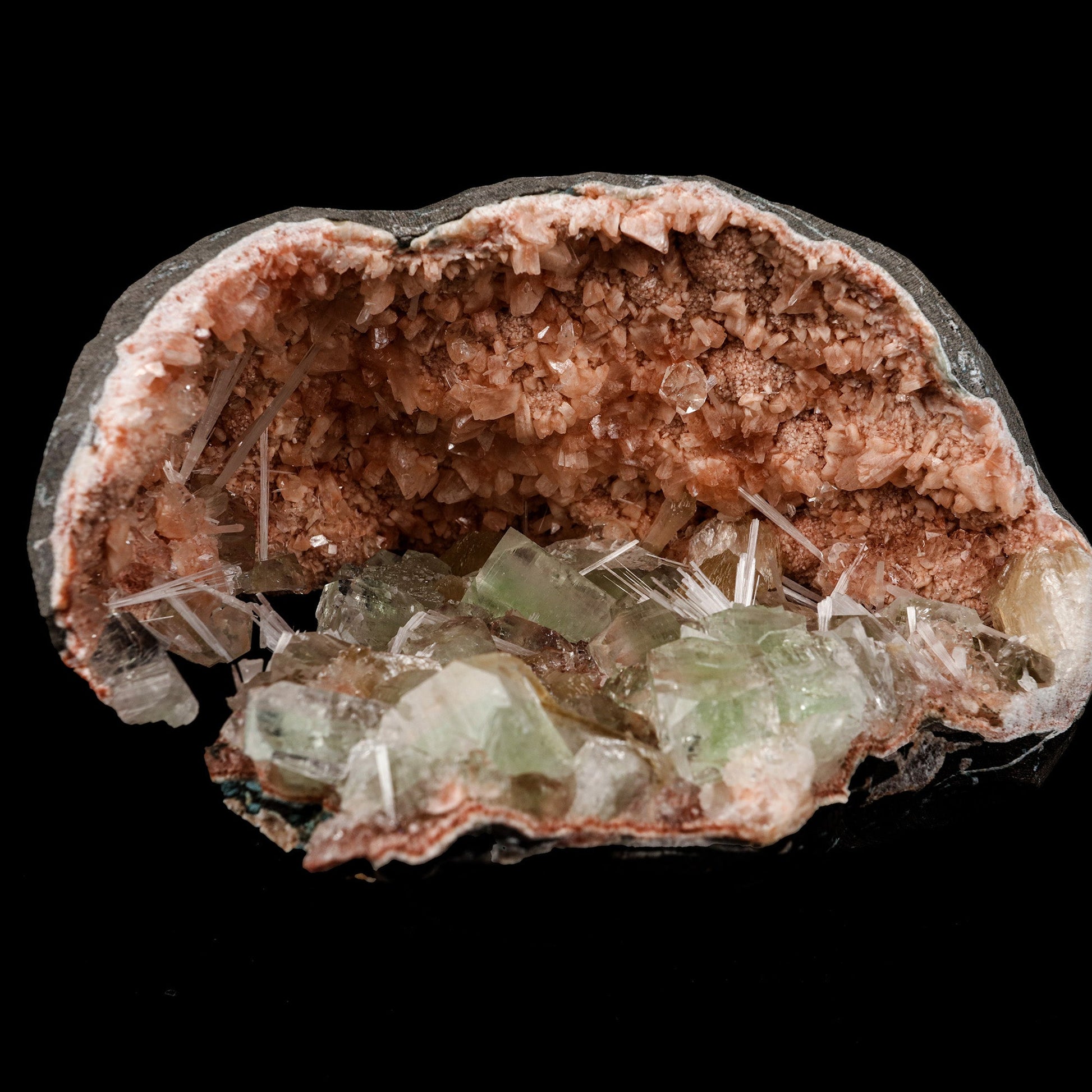Against a black background, an oblong-shaped rock, resembling ordinary gray granite, has been meticulously cut in half, revealing its hollow interior brimming with crystalline structures. The outer surface of the rock is a solid dark gray, contrasting starkly with the vibrant formations inside. Predominantly, small, reddish-brown crystals densely cluster in the center and upper part of the exposed section, giving off a pinkish-red hue. These crystals dominate the interior landscape. In the lower portion of the rock, large, greenish-white crystalline structures catch the eye with their translucent quality, resembling long, fibrous strands akin to fiber optics. The combination of reddish-brown and greenish-white crystals, set against the gray rock and black backdrop, creates a visually striking geologic mosaic.